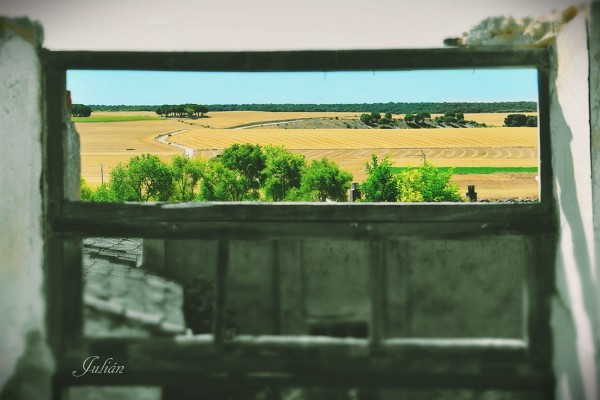The image is a photograph capturing a picturesque window view set into a dilapidated white painted wall, missing its roof. The old, rotting wooden window, devoid of its glass panes, reveals a detailed scene of the outside world. In the foreground, directly through the lower half of the window panes, the monochrome gray shingles on the lower part of the building's roof can be seen. Beyond this foreground, the landscape unfolds with multiple trees laden with green leaves, which precede expanses of well-kept yellow fields designated for farming. A thin river meanders through these fields, contributing to the idyllic rural setting. In the far distance, a hill covered with trees rises slightly, adding depth to the serene vista. The sky above is a clear, light blue with no clouds, indicating a calm daytime atmosphere. In the lower left corner of the image, the name "Julian" is inscribed in white cursive text, likely attributing the work to the photographer or artist.